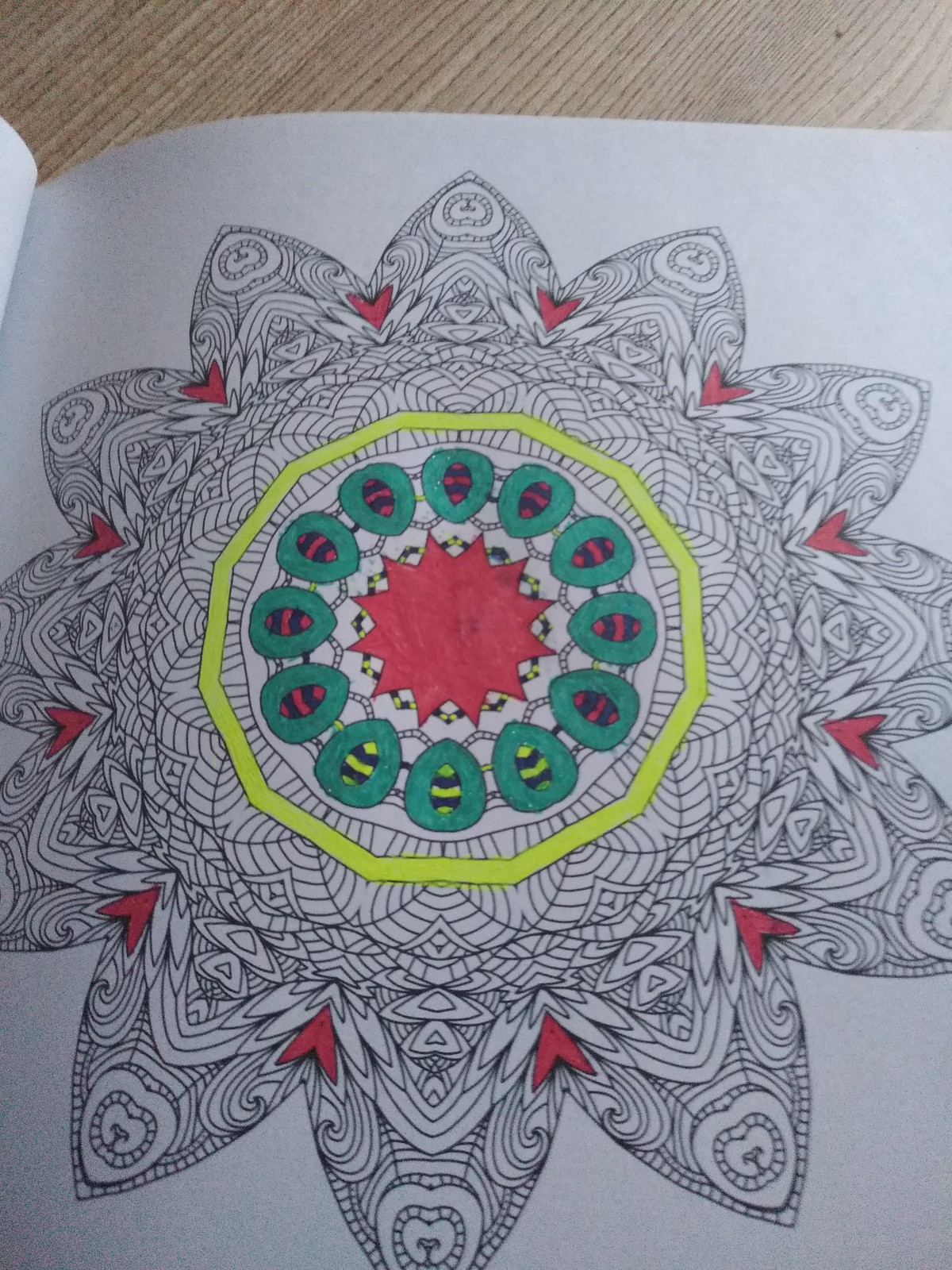The image features a vertically aligned rectangular page from an adult coloring book, partially open. In the upper left-hand corner, the book’s crease is slightly visible, indicating the edge of the page. The primary focus is on a detailed mandala design, resembling a sun or a flower, with intricate layers and patterns comprising petals and diverse shapes. The page displays partially completed coloring, where the artist has meticulously colored small red hearts in one of the layers, a yellow rough-edged circle surrounding a section, and teal hues on leaf-like structures. Additionally, red and black elements are filled in within the center along with a red star. This work-in-progress is set against the backdrop of a brown table, providing a warm and rustic contrast to the vibrant colors.